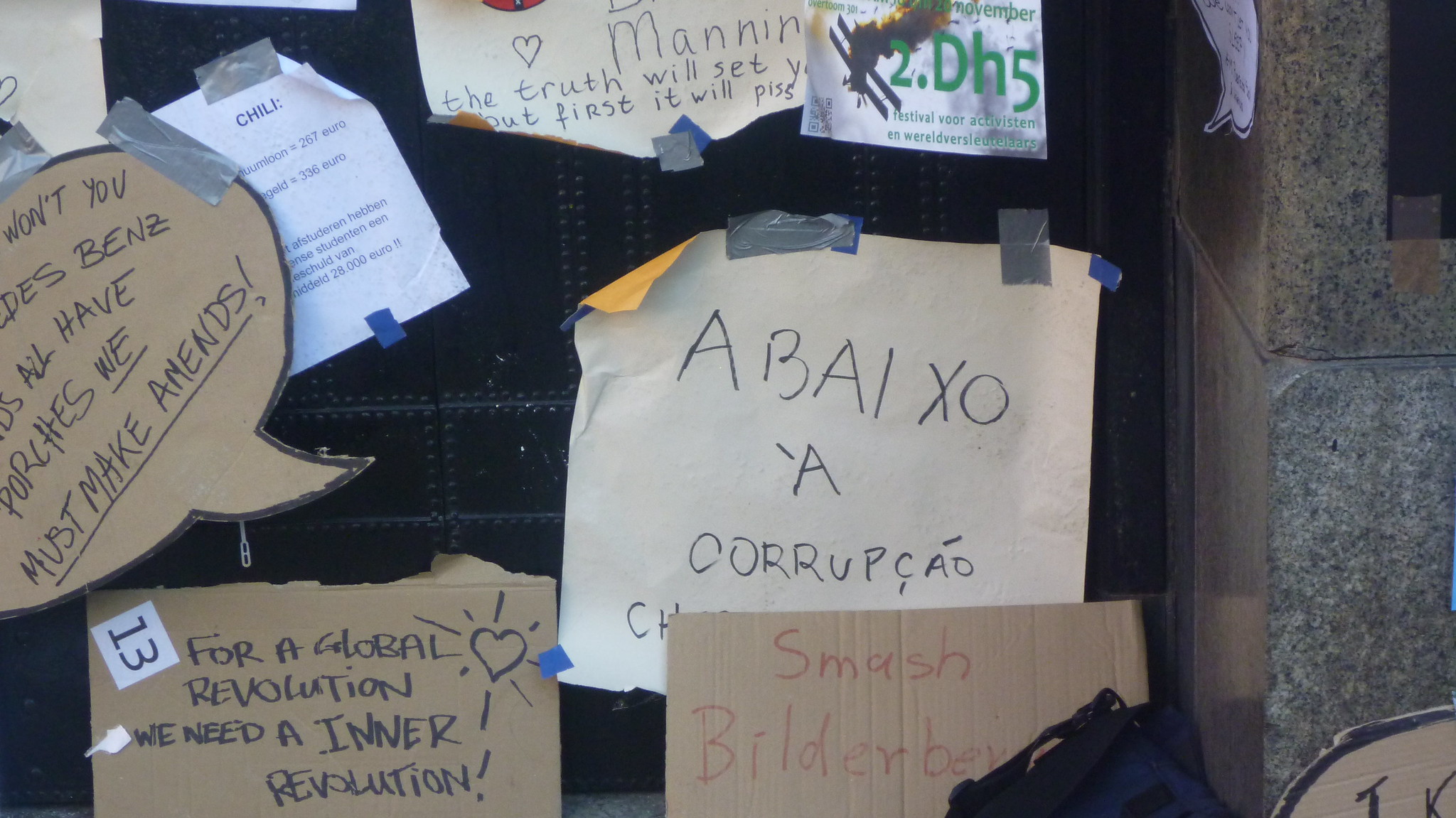This wide rectangular image captures a wall of diverse posters. The surface is predominantly black, speckled with evenly spaced black dots, and on the right, the corner of the wall is made of dark gray speckled marble bricks. In the center-right, there's an off-white piece of slightly bent paper taped on, reading "ABAIXO A CORRUPÇÃO" in black ink. To the left of this, a sideways speech bubble sign with all capital letters is partially visible.

In various parts, note cards crafted from cardboard and paper are affixed to the wall, some secured with duct tape. The lower left corner features a cardboard sign with the text, "For a global revolution, we need an inner revolution," accompanied by a heart symbol and the number 13. Nearby, another cardboard sign bears the phrase "Won't you, Des, Benz, all have Porsches, we must make amends," though it is partially cut off in the image.

Positioned on the right lower side, a cardboard poster declares, "Smash Bilderberg," penned in red text. Other messages, such as "The truth will set you free but first it will piss" and another one reading "chili" accompanied by some numbers, are scattered throughout. Notably, a backpack rests on the ground in front of some of these signs, further indicating a scene of impromptu, expressive documentation.